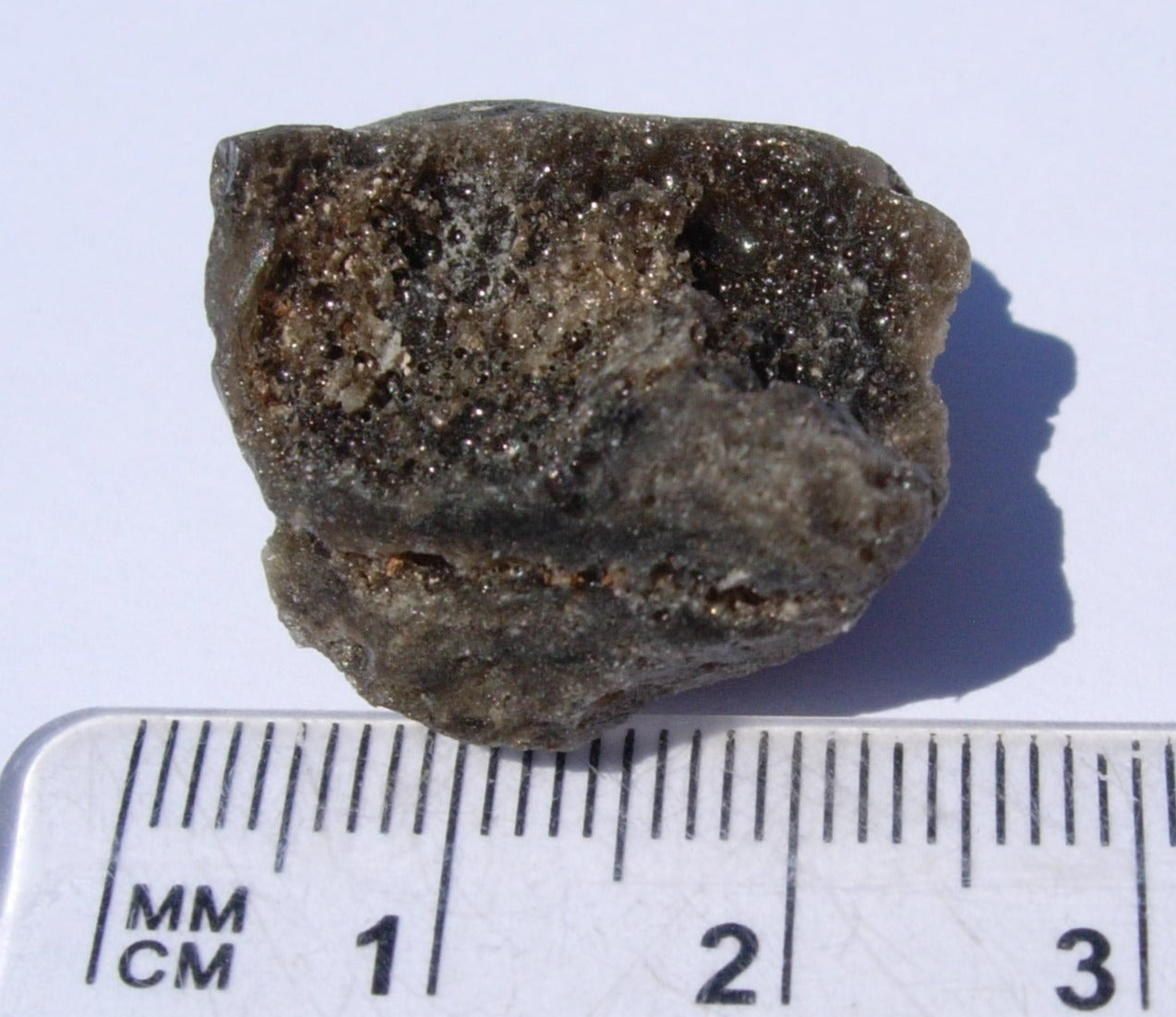An up-close, detailed image shows a jagged, porous rock specimen with intricate indentations and a mixture of dark colors such as black and dark gray, interspersed with flecks of gold, cream, and white. The rock rests on a light purple background, casting a clear shadow to its right due to the overhead light. Below the rock, a transparent ruler marked in millimeters and centimeters stretches from the left side of the image. The ruler has black numbering visible from 1 to just over 3, with the left side labeled "MM" and "CM" in capital letters. The rock appears to measure approximately two and a half centimeters in length, aligning with the ruler for scale.